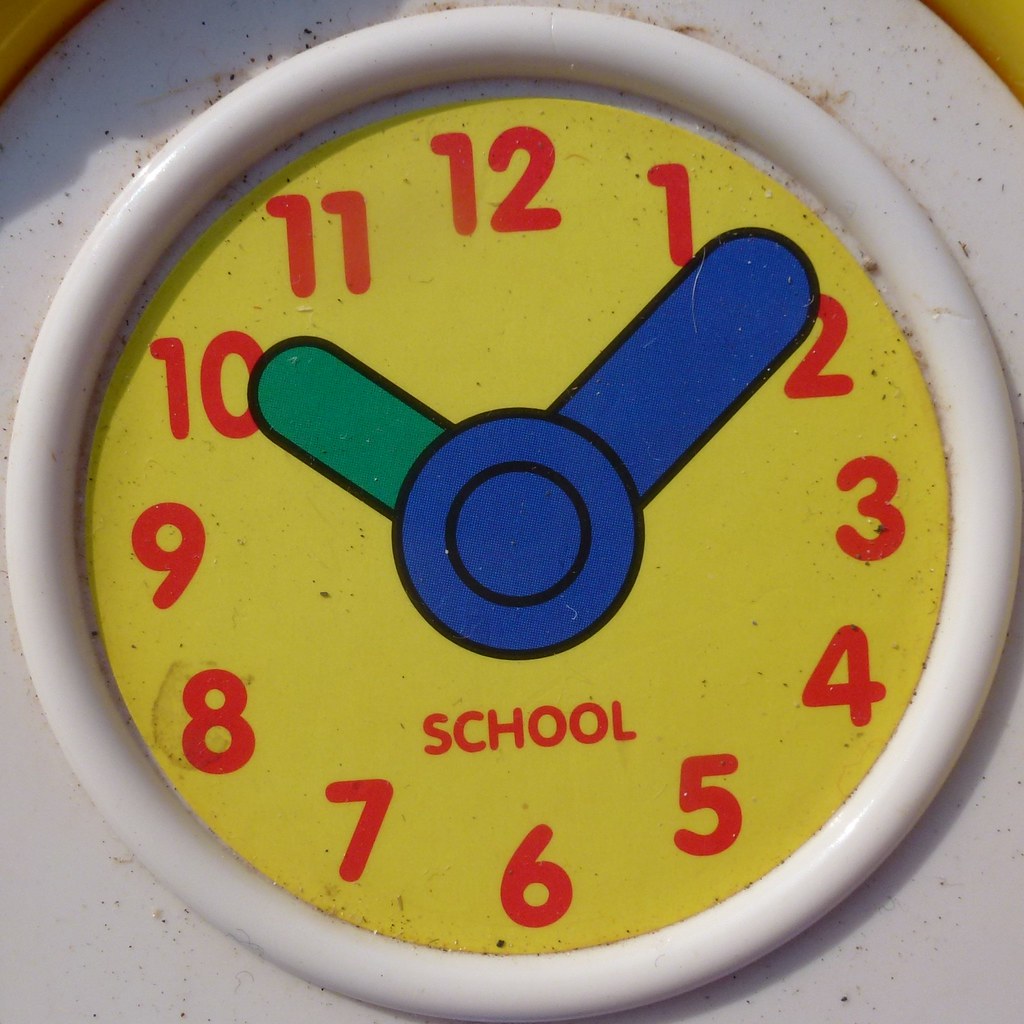This is an image of a children's school clock set against a mixed yellow and white background. The clock features a vibrant face with numbers 1 through 12 clearly marked. The hour hand is depicted in green, while the minute hand is shown in blue. The clock has the word "school" prominently displayed on its face in red text. The colorful design and clear numbering make it an effective educational tool for children learning to tell time.